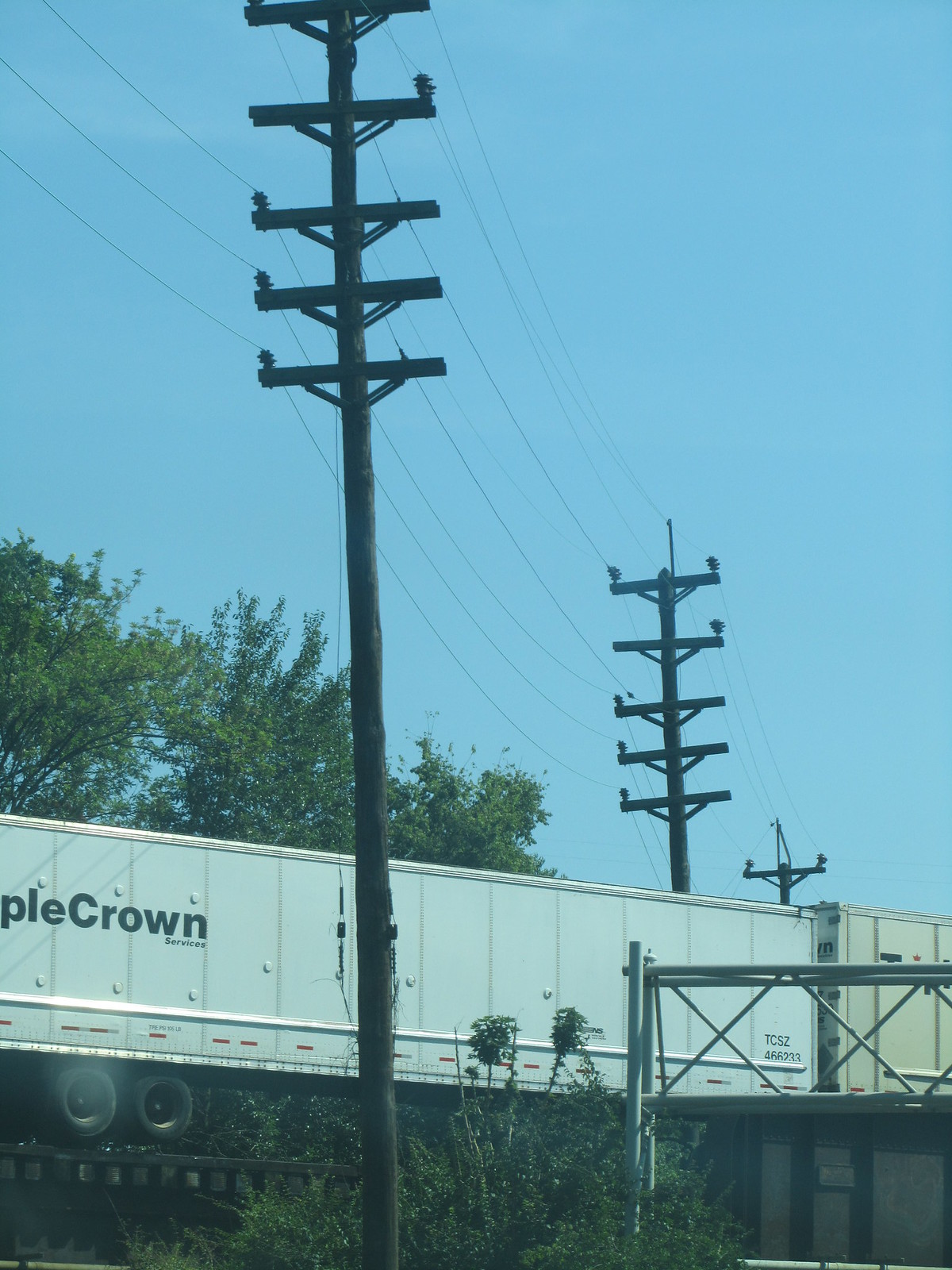The image features an elevated train track carrying a long, white cargo train car marked with the partially visible word "P-L-E" followed by "CROWN," with the "C" being capitalized but the entire word still merged. Beneath the "W" and "N" of "CROWN," the word "services" is written. The train car has registration number T-CSZ 466-233 and is seen against a blue sky backdrop punctuated by scattered leaves and three tall electrical poles. These poles carry multiple thin wires, stretching  between them. In the left corner, tall trees are visible, with bushes and greenery sprawling at the bottom of the image. There is a fence area to the right of the photo, adding to the rustic, elevated woodland scene. Additionally, five wooden beams, each about 10 inches long, are secured to the top of the electrical poles, with the poles themselves extending upwards in different stages of elevation, creating a network of wires silhouetted against the clear sky.